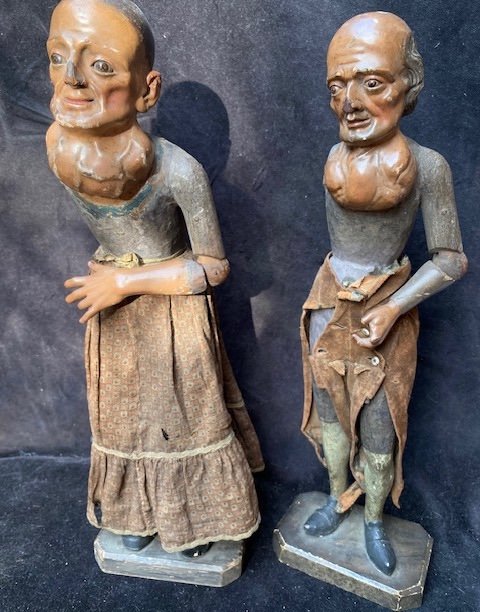The vertically rectangular, full-color photograph, which appears to have been staged indoors, features a pair of eerie, intricately carved statues of a man and a woman standing on a rectangular pedestal against a bluish-gray background. The statues, which bear a semblance to wooden dolls, exhibit unsettling facial features, including large, bizarre growths resembling sacks under their chins. The woman wears a blue top and a brown dress extending to her ankles, and the man beside her, who is balding with sparse gray hair at the back, is clad in a grayish-blue top, blue pants, and dark blue shoes, with a tattered brown garment around his waist. Both figures appear to have been restored, indicating signs of past deterioration. Their presence and condition lend an air of antiquity and melancholy to the scene, further accentuated by the unsettling, decayed appearance of their faces.